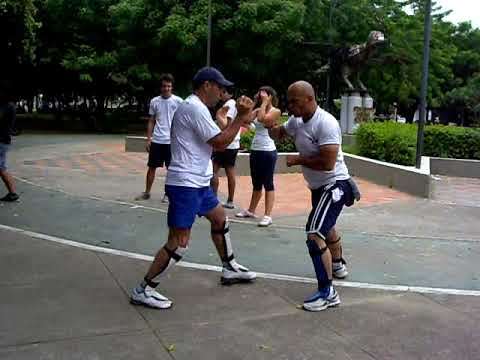In this detailed outdoor scene, two African American men, both clad in white t-shirts, blue shorts, and knee pads, are standing on a gray pavement, seemingly pretending to fight or spar with each other. Both men are of medium build and height; one is sporting a blue cap and the other has very short hair. They also have white sneakers on, and their hands are raised as if they are practicing fighting techniques. 

Behind them, there's a mix of spectators, including a woman in a white tank top and blue shorts, and two men also dressed in white t-shirts and blue shorts. Another person stands further back, wearing a black shirt and blue jeans. Additionally, a girl with her hands over her eyes in disbelief is seen observing the scene.

The background showcases a town-like atmosphere with a circular walkway and painted brick detailing, blending into a green area filled with numerous trees. A statue, resembling a dinosaur made of bronze, is discernible, hinting at a park setting. Light poles, likely street lamps, are spread throughout the area, and the entire scene is illuminated by daylight.